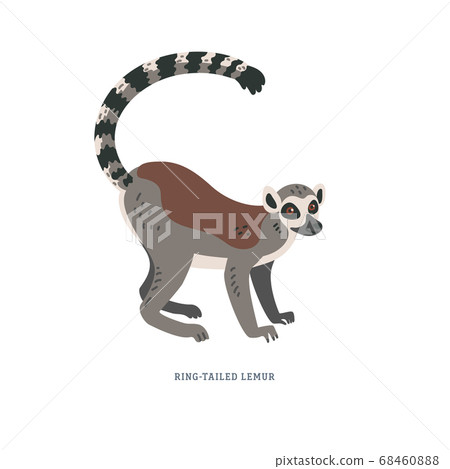This detailed stock photo features a ring-tailed lemur set against a minimalist white background with faint gray lines forming a large X pattern, converging at the center where the animal is positioned. A watermark icon with the word "PIXTA" in gray letters is also centered on the image. The lemur is captured in a right-side profile with its face directed to the right.

The lemur's facial features are distinct: it has a stark white mask around its striking eyes, which are a deep reddish-brown surrounded by black rings. Its ears are white on the edges with dark black interiors. The nose is gray, and the forehead displays speckles of gray. The head is gray, and its snout is black, adding to its distinct facial characteristics.

The lemur's body presents a mix of colors and textures. The top or back of the body is a coffee brown color with a somewhat splotchy appearance, while the sides, legs, and lower body are gray. The belly and neck area are cream or white. Notably, the two legs on the left side are a darker gray compared to the lighter gray legs on the right side.

Its iconic tail, which curves upwards towards the upper left corner of the image, features a striking black, white, and gray striped pattern with a ruffled black tip. Underneath the animal, the text "ring-tailed lemur" is inscribed in gray letters, identifying the species.